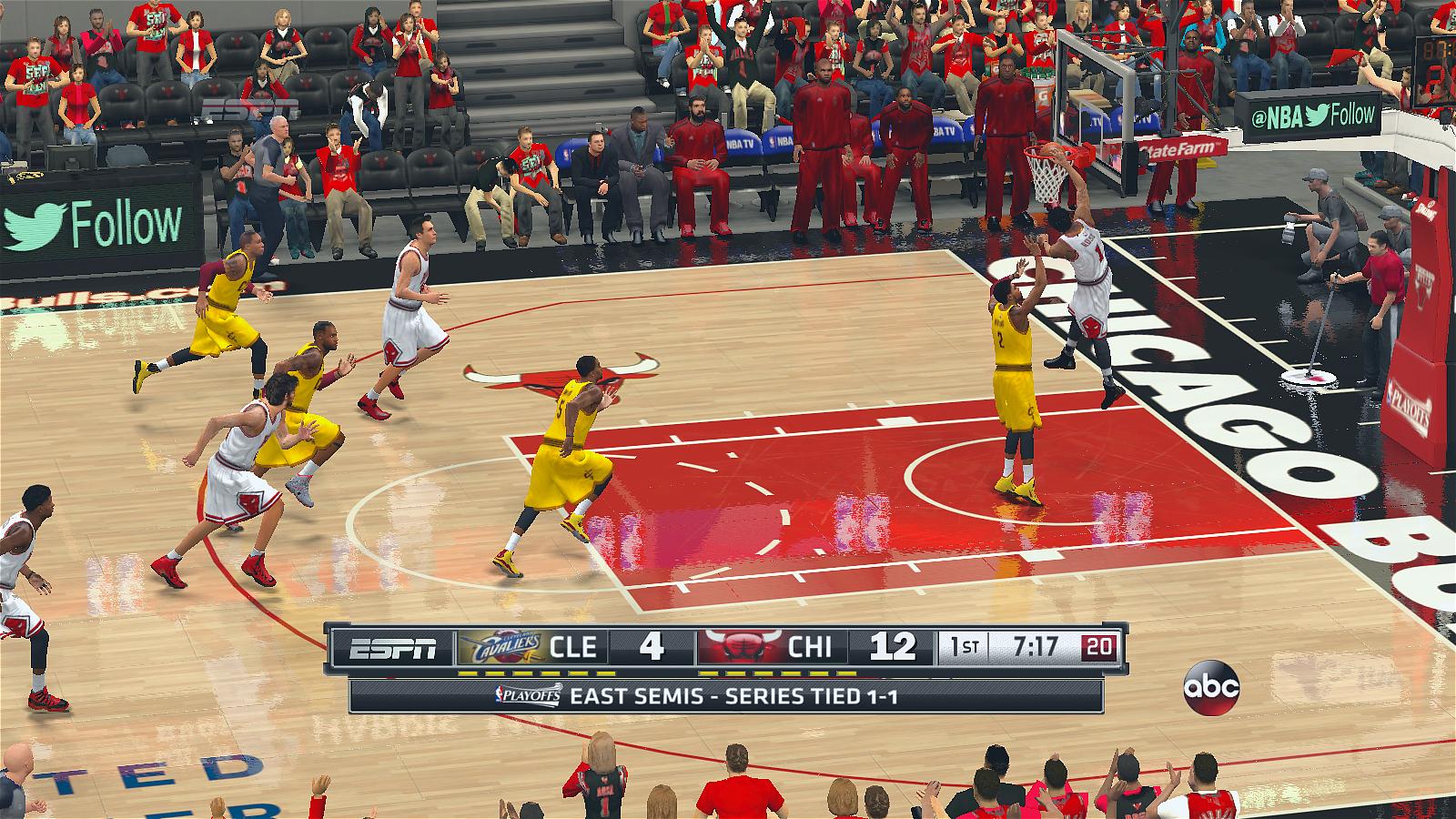A highly realistic screen capture of an intense playoff basketball game between the Chicago Bulls and the Cleveland Cavaliers is displayed in a horizontal format. The scene is set on the iconic Chicago Bulls court, where players from both teams are captured in the heat of action. The Bulls, dressed in their traditional white uniforms, are up against the Cavaliers, who sport striking yellow uniforms with red numbers. 

At the focal point of the image, Bulls' player number 1 is executing a powerful dunk over a towering Cavaliers defender. The dynamic moment is framed by an engaged crowd, with fans energetically cheering from the stands. On the sidelines, both teams have several players seated on their respective benches, intently observing the game. 

Prominent Twitter promotional signs are visible in the background, urging fans to "Follow" and "Follow @NBA" alongside a "State Farm" advertisement. The scoreboard reveals that the Bulls are leading the Cavaliers 12-4 with 7:17 remaining in the first half. This pivotal game is part of the Eastern Conference Semifinals, with the series currently tied at 1-1, heightening the stakes for both teams as they vie for dominance.